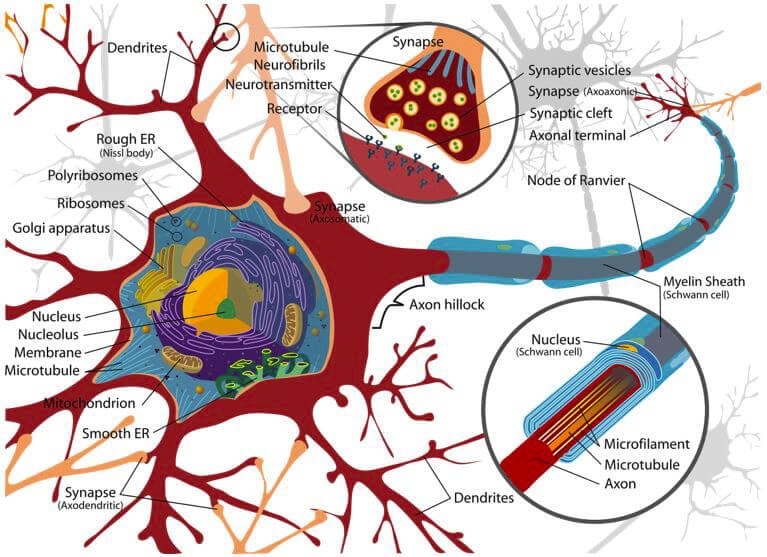This image, likely from a textbook or research paper, intricately details the structure of a nerve cell (neuron). The main part of the cell is highlighted in red, with additional components depicted in blue. The neuron is extensively branched, characteristic of its function. Key parts of the neuron labeled in the image include the nucleus, nucleolus, membrane, mitochondrion, rough ER, smooth ER, Golgi apparatus, ribosomes, and polyribosomes. Noteworthy structures such as the axon hillock, dendrites, synaptic vesicles, synapses, axon, and the node of Ranvier are clearly marked. Close-up views are provided for the synapse and nucleus, with parts illustrated in various colors like purple, orange, and green. The diagram is densely annotated, with arrows pointing to each organelle and cell part, making it a comprehensive visual guide to the neuron's anatomy.